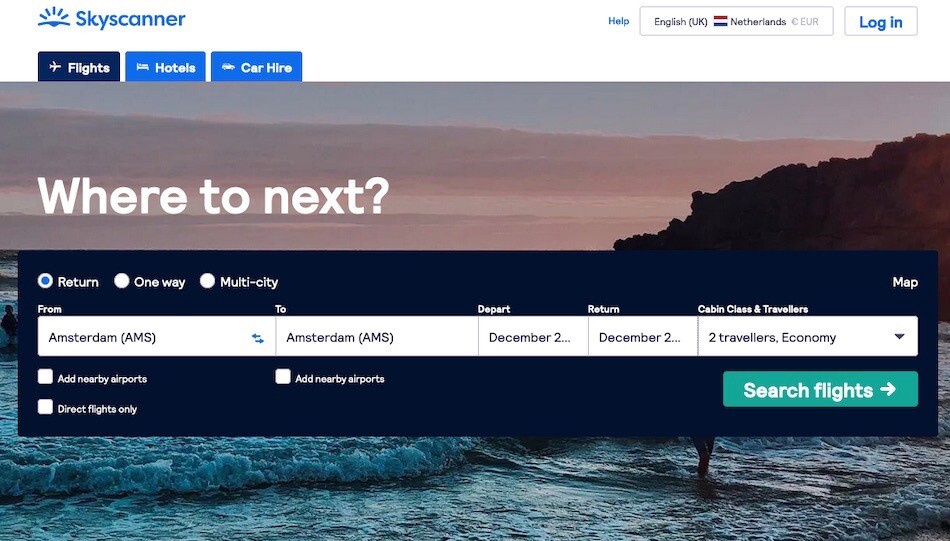This screenshot from the Skyscanner website showcases a comprehensive travel planning interface where users can book flights, hotels, and rental cars all in one place. At the top left, the Skyscanner logo is prominently displayed, while a "Help" option is conveniently positioned on the top right.

Below, there's a main selection box where users can set their departure and arrival destinations. In this instance, the interface shows "English (UK)" and the Netherlands flag with "Netherlands" next to it. The currency displayed is the British pound symbol followed by Euros. Adjacent to this box is a smaller "Login" button in blue text.

Beneath the main selection area, users can explore categories for flights, hotels, and car hire, adapting the interface to their needs. The central image features a serene beach scene with a few people and rolling waves, framed by cliffs in the background. Superimposed on the image is the text "Where to next?" in white.

Further below, travelers can input detailed trip information such as departure and arrival locations, departure and return dates, and the number of travelers. In this example, the trip parameters are set with two travelers economy class traveling from and to Amsterdam, with unspecified dates indicated as "December 2..." for both departure and return. Additional options including "Add nearby airports," "Direct flights only," and another "Add nearby airports" are not selected. A clickable "Search flights" button is available for users to proceed with their travel search.